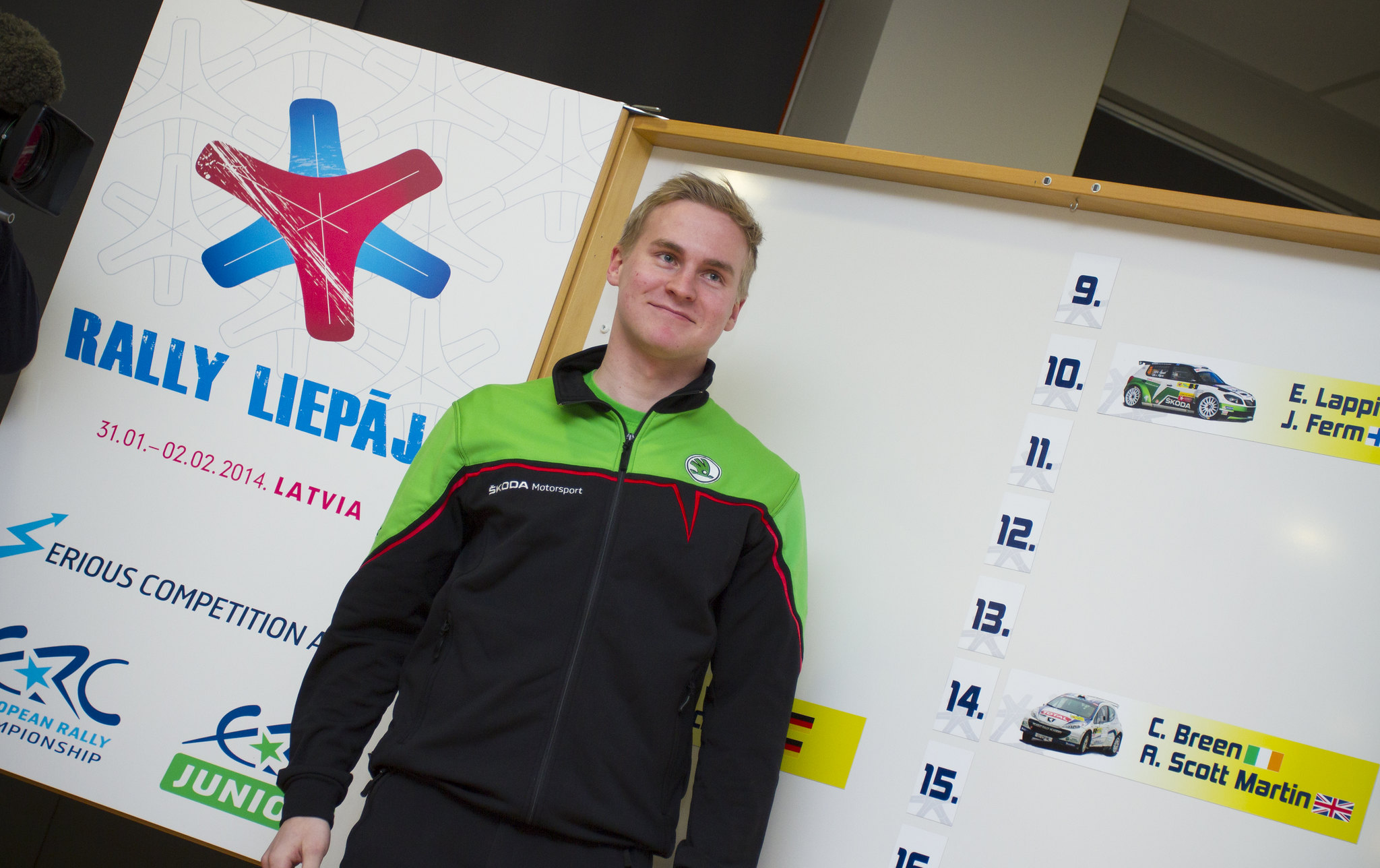The image shows an indoor setting in what appears to be a competition hall, characterized by visible walls, ceiling, and pillars in the background. There's a prominent bulletin board on the left side with a poster board next to it, displaying the text "Rally Lepa" alongside a date "31-01-22-2014" and mentioning Latvia and the "Eris Competition." A Caucasian gentleman with short strawberry blonde hair is standing in front of the display, wearing a black and neon green racing jacket bearing the ŠKODA logo and "ŠKODA Motorsport" inscription. He appears a bit shy and was possibly not expecting to be photographed. To his right, there's a scoreboard listing the numbers 9 through 16, where numbers 10 and 14 have car images and driver names next to them. Number 10 lists "E. Lappi J. Firm," and number 14 lists "C. Breen R. Scott Martin," with adjacent country flags. A distinct banner with a blue and red star logo, indicating sponsors from the European Rally Championship Junior, is also visible.